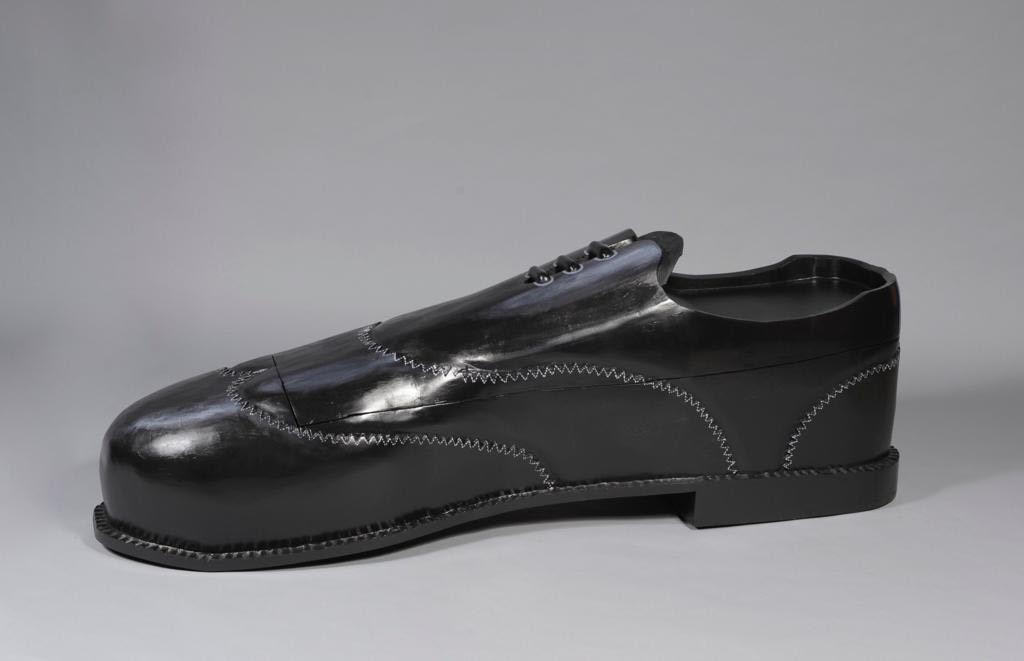The photograph features a meticulously crafted black shoe, reminiscent of a man's dress loafer, displayed against a seamless light gray backdrop, suggesting a professional photography setting. The shoe, made of a shiny material, possibly painted, reflects light, showcasing its polished surface. It is not functional as it appears solid and filled with the material it is carved from, resembling wood or perhaps another substance, despite the presence of realistic shoelaces. Distinctive white stitches zigzag around the shoe, with three sets visible on the front and along the low back, emphasizing its detailed craftsmanship. The elongated toe area and rounded tip give the shoe a slightly unconventional appearance. The slightly raised heel and overall design suggest a traditional men's low-heeled, black church shoe.